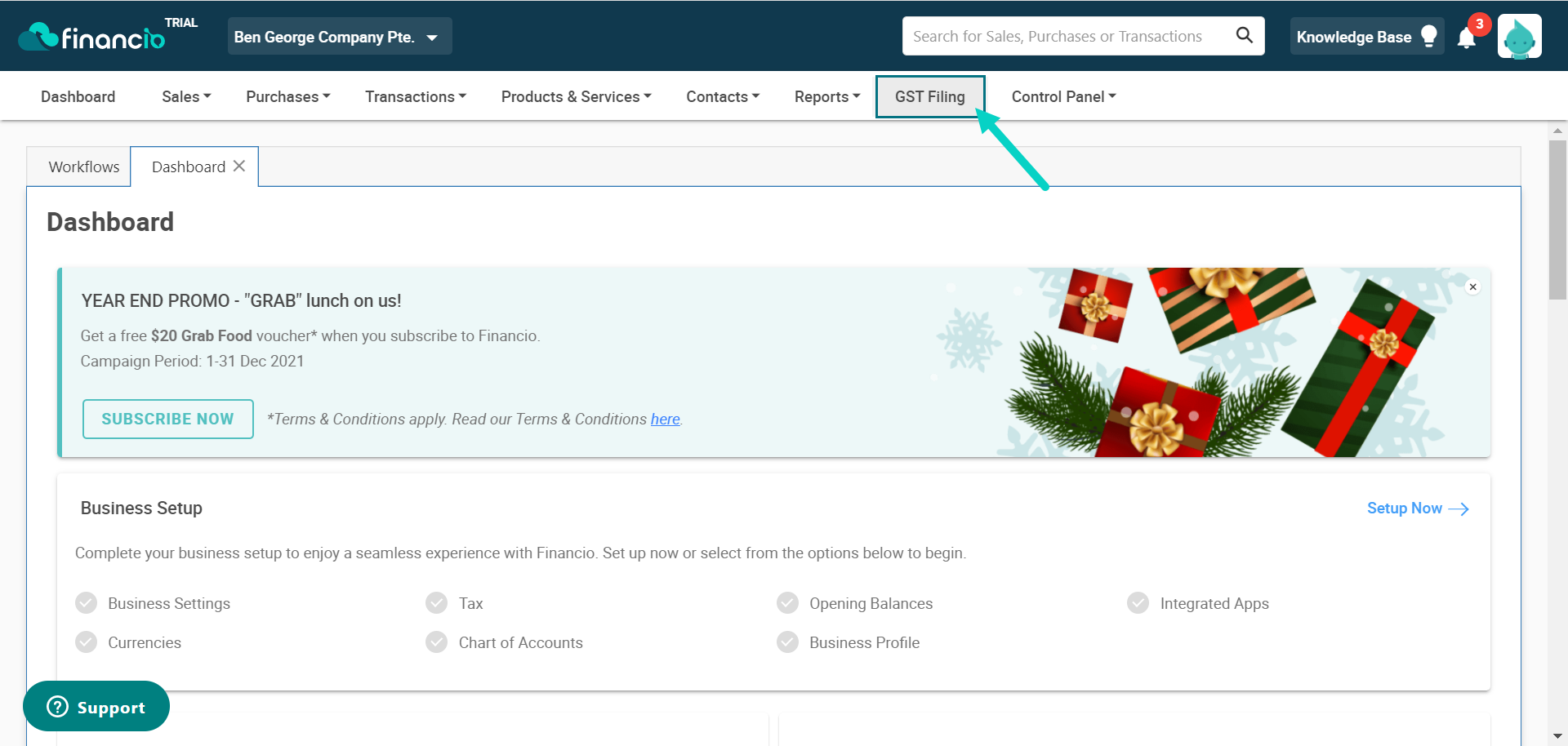The image consists of a user interface featuring a blue header with the logo "Financio." The "IO" in the logo is highlighted in blue. Adjacent to the logo, there's a "Trial" label and the text "Ben George Company Pro." Below the header, a search bar is present alongside a "Knowledge Base" icon depicted by a light bulb. Additionally, there's a notification symbol indicating three new notifications and an icon resembling the Reddit logo.

The left sidebar menu includes options such as:
- Dashboard
- Sales
- Purchases
- Transactions
- Products and Services
- Contacts
- Reports
- GST Filing (highlighted in gray and outlined in a blue rectangle with a blue arrow pointing to it)
- Control Panel

Within the dashboard, a selected white rectangle bears the text "Windows Dashboard." A promotional banner at the top mentions "Year-End Promo: 'Grab Lunch on Us'!" enclosed in quotation marks. There is also a call-to-action blue rectangle labeled "Subscribe Now" in blue text. Below this, there is a note reading "Terms and Conditions Apply. Read our terms and conditions here," with "here" being a clickable hyperlink.

An image of Christmas presents decorates the interface, indicating a festive theme. Additionally, there's a "Business Setup" section with a "Setup Now" button in blue coupled with a rightward arrow. A prompt encourages users to "Complete your business setup to enjoy a seamless experience with Financio."

Overall, the interface is visually structured and user-friendly, emphasizing key functions and promotional offers while guiding users through business setup and navigation.